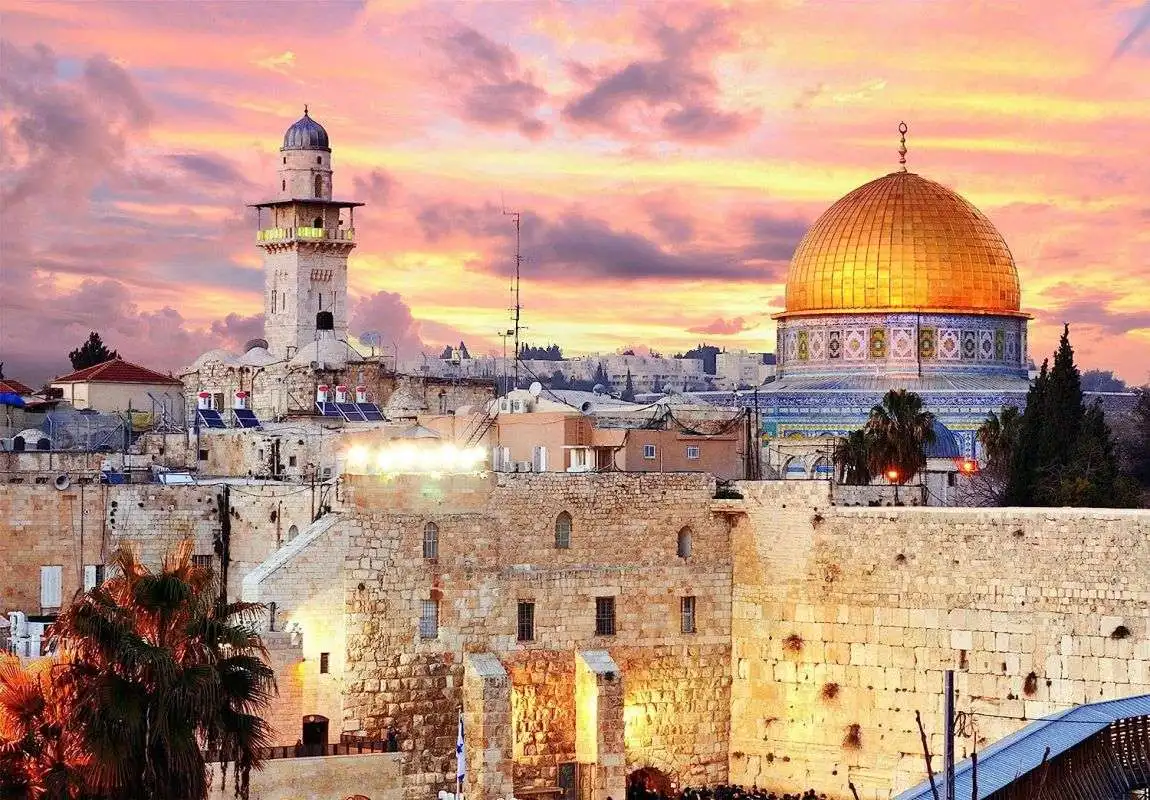The photograph captures an urban view in the Old City of Jerusalem, featuring a landscape of tan stone buildings. Dominating the scene towards the back right is a tall, lighthouse-like structure with a blue dome at the top and a small square outcropping below that. This structure has a wide base with metal stairs leading up. Central in the frame is the iconic Western Wall, or Wailing Wall, partially visible from a vantage point on the ramp leading to the Temple Mount.

To the right, the magnificent Dome of the Rock stands out with its gold-tiled dome adorned with diamond shapes at the base and beautiful blue mosaic work. This domed structure, amidst its Islamic architectural charm, reflects the hues of a setting or rising sun, casting pinks, yellows, and purples across the sky. Street lights flicker on, mingling with the natural twilight, and a few trees dot the Temple Mount. The skyline includes satellite dishes, solar panels, and additional buildings fading towards distant apartment blocks on a further mount.

In the foreground, one can spot palm trees adding a touch of greenery. The scene is lively, with groups of people gathered at the Western Wall, enveloped in the historical and spiritual ambiance that the city exudes.